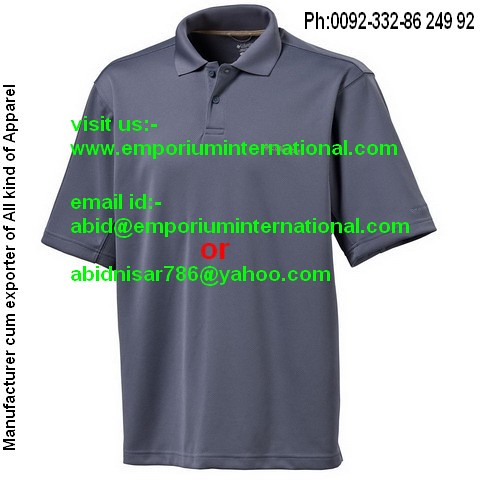The image is an advertisement for a clothing website featuring a gray short-sleeved collared shirt with a white lined collar and two buttons, with the first button open. The shirt sits at a slight angle on a white background. In the top right corner, there is a phone number in black text reading "PH 0092-332-8624992." Along the left side, written vertically in black text on a white background, it says, "Manufacturer come exporter of all kind of apparel." Across the chest area of the shirt, green text horizontally states, "Visit us: www.emporiuminternational.com," followed by "Email ID: abid@emporiuminternational.com," and then "or" in red, with the alternative email "abidnissar786@yahoo.com" in green.